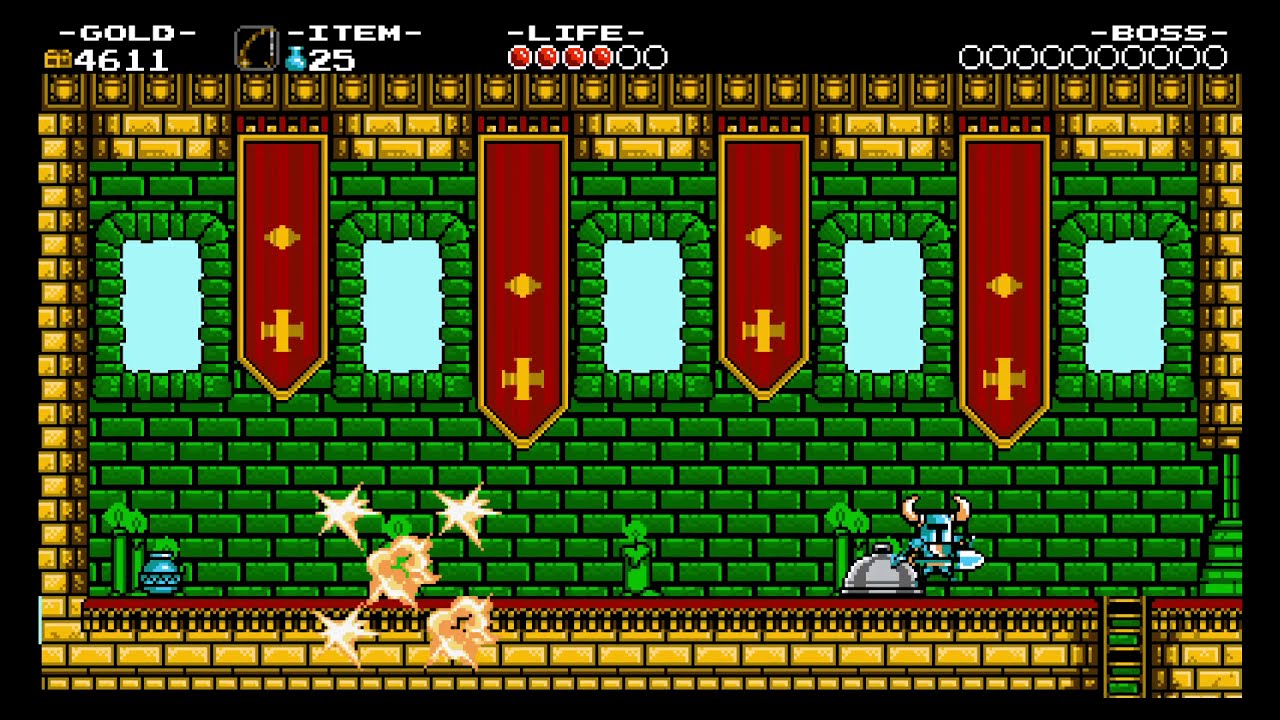This image is a screenshot from an older, pixelated video game with a medieval theme. The central playing area is composed of green bricks with small portals interspersed between them, and framed by yellow bricks. Against this green brick wall stands a knight-like character clad in blue armor, complete with Viking-style bull horns on its helmet. Adjacent to the character is a blue pot and several glowing green candles.

At the bottom right of the image, the knight stands near what appears to be a dome with a service tray, hinting at an interactive object or power-up. Meanwhile, the lower left corner reveals multiple small explosions, indicating the area has been struck by shells or projectiles.

Overlaid across the top of the image are various game stats and interface elements, starting with the word "gold" followed by the number 4611. Further to the right is the word "item" accompanied by the number 25 and an image of a blue vase, then the word "life" with four out of six red indicator dots lit up, representing the player's remaining lives. To the far right, the word "boss" is displayed above several zeros, possibly related to a boss battle progression or countdown.

Additionally, there are flags with cross and diamond patterns in gold at the top of the screen, and pools of water can be seen between these flags, contributing to the rich, albeit simplistic environmental detail of the game.